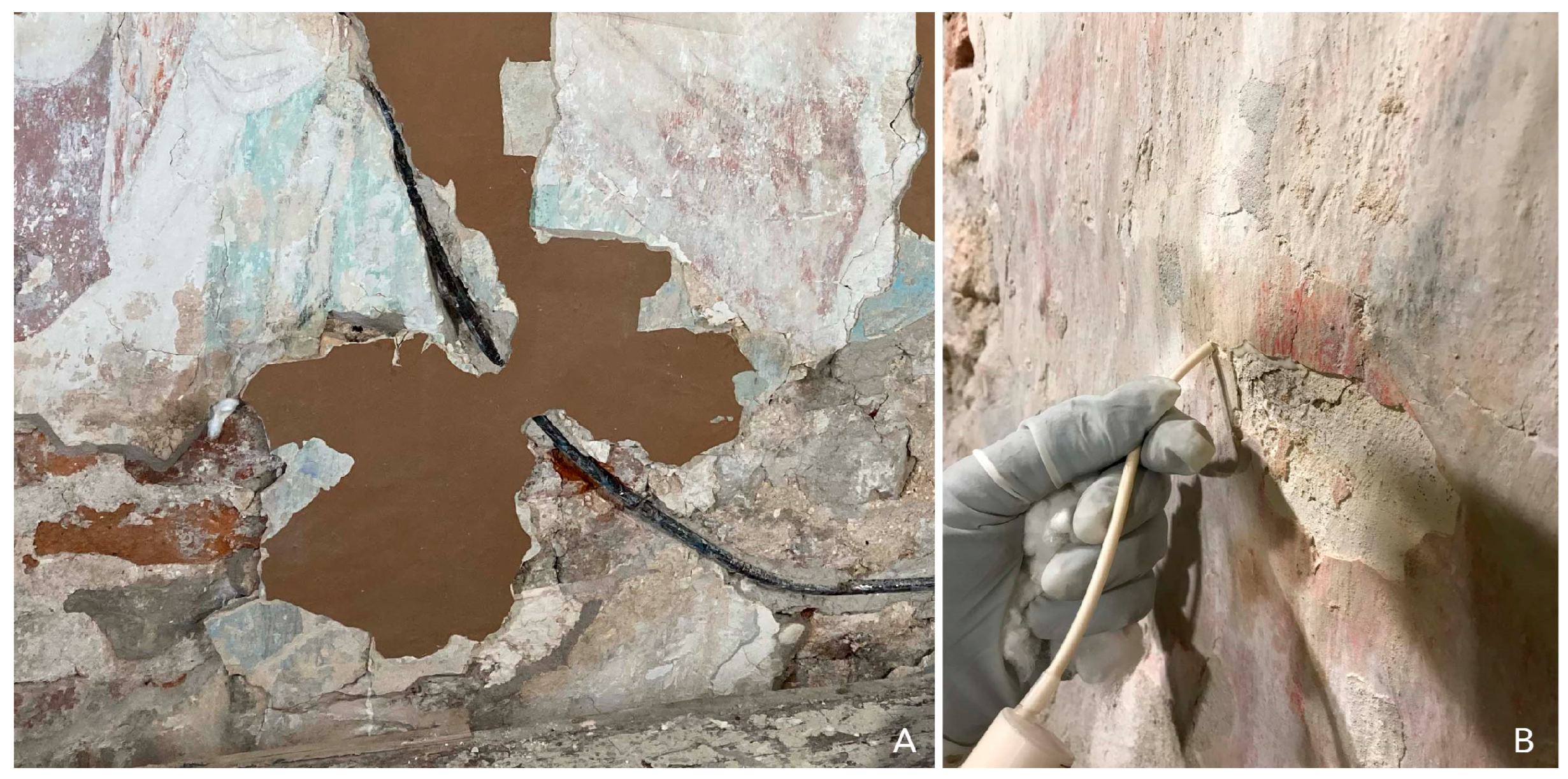The split image features two side-by-side photographs labeled "A" and "B," showcasing a wall undergoing restoration. The left photograph, marked with a capital "A" in the bottom right corner, displays a dilapidated wall with peeling paint and visible cracks. The wall's rough surface reveals an irregular section in the center, coated with a medium brown substance, suggesting prior repair work. The wall exhibits lighter hues of white and light blue surrounding the brown area, hinting at its original painted condition. A cable-like image painted on the wall adds to its weathered appearance.

On the right, the photograph labeled "B" presents a close-up of the same damaged wall, but with a discernible restoration effort in progress. A gloved hand, holding a thin, ivory-colored tube, extends from the left side of the image. The tube's end appears to be used to apply some sort of filling material to the wall, signifying the restoration process aimed at mending the cracks and peeling sections. The gloved hand and the tool highlight the meticulous work being undertaken to restore the wall's surface.